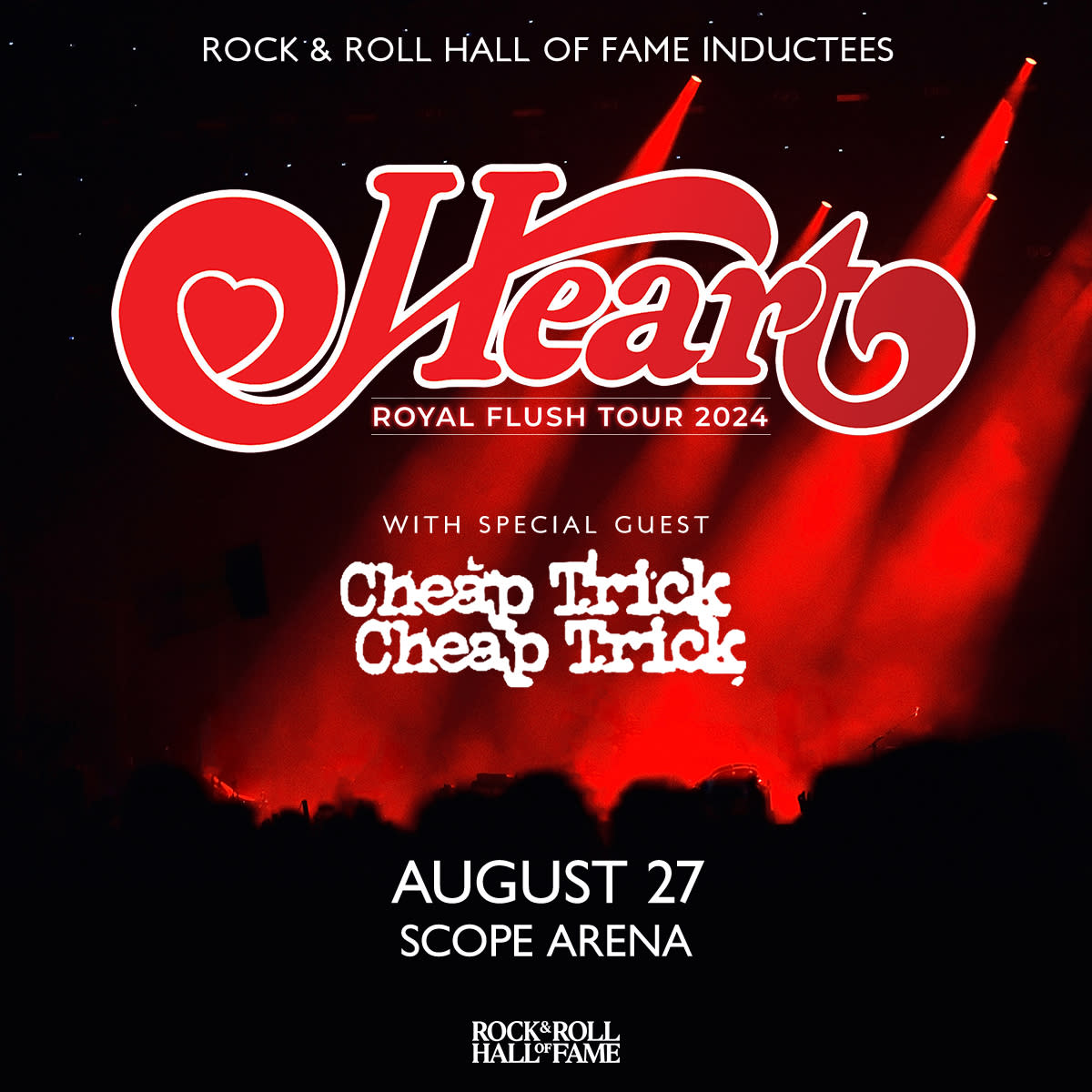The poster is a sleek advertisement for a rock concert event titled "Heart," part of the Royal Flush Tour 2024. The background is predominantly black, providing a dramatic backdrop that accentuates the vibrant colors used in the design. At the top of the poster, in bold white lettering, it prominently announces "Rock and Roll Hall of Fame Inductees." Below this, the name "Heart" is strikingly displayed in modern red script with a heart graphic elegantly integrated into the first letter. Following this, in pink print, it reads "Royal Flush Tour 2024."

Just beneath, the text highlights the special guest, "Cheap Trick," written in a unique and eye-catching font. Further details include the event date, "August 27th," and the venue, "Scope Arena," both in white text. Red spotlights and faint red smoke add a dynamic and energetic feel to the black background, making the poster visually compelling. Additionally, a white outline enhances some of the central elements, adding to the overall modern aesthetic of the design. This event is clearly presented as a significant one, sponsored by the Rock and Roll Hall of Fame, emphasizing its prestige.